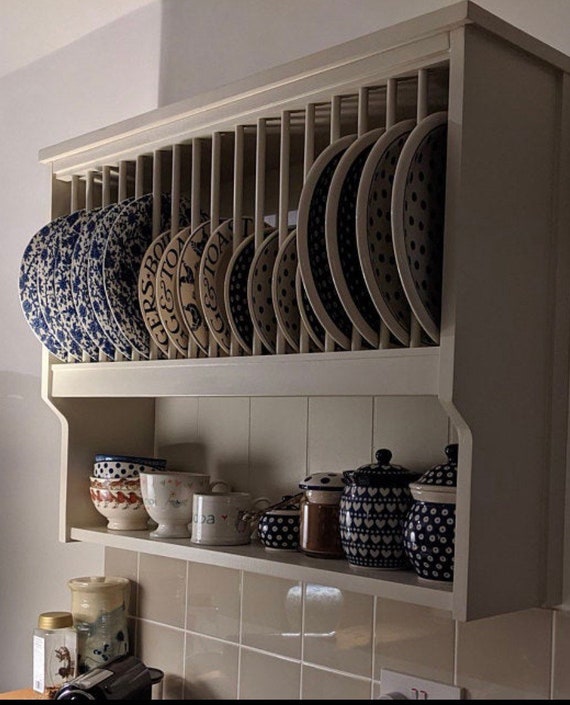The image showcases a section of a kitchen interior highlighting organized storage and design elements. In the upper third of the image, a hanging cabinet with two shelves is seen. The top shelf features a plate rack with blue and white plates of various designs and sizes: six or seven flowered plates on the left, four plates in the center with some text like "CERS" or "GERS," three smaller plates to the right of center, and four large plates on the far right, all with blue embellishments such as flowers or dots. Below this rack, occupying the middle third of the image, the shelf contains an assortment of cups, including soup bowls and a coffee mug or creamer, along with jars possibly holding sugar, salt, and other kitchen essentials. The bottom third of the image displays a tile backsplash with additional jars in the bottom left corner and an electrical outlet on the right side. The kitchen exudes a cozy style with a color palette of blue, white, brown, tan, and gray.